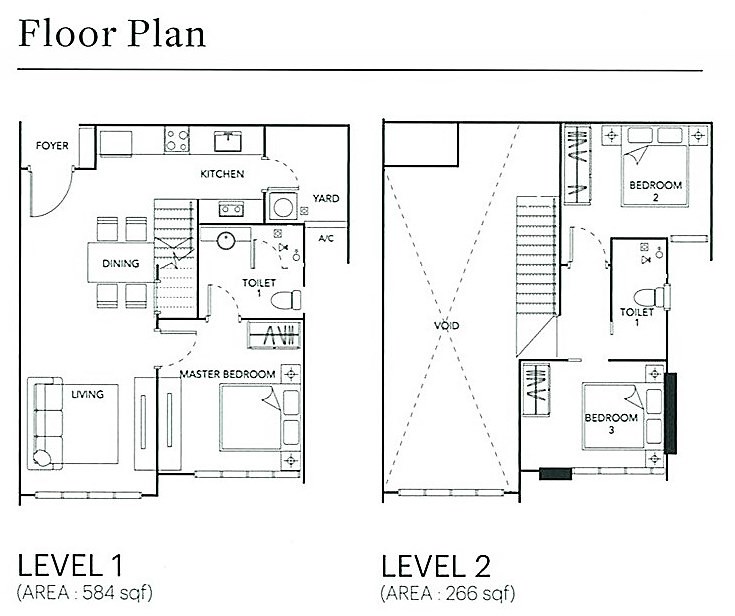This detailed black and white architectural print illustrates the floor plan of a two-story residential space, displaying measurements and layout for both levels. The left side features the detailed layout of Level 1, labeled "Level 1 (Area 584 square feet)" at the bottom. Upon entering through the front door, you step into a foyer that leads directly to the kitchen, where the stove, sink, and refrigerator are meticulously drawn. Adjacent to the kitchen is a dining room, followed by a staircase leading to the second floor, a toilet, a full bathroom, a spacious living area, and the master bedroom. 

On the right side of the print, Level 2 is displayed, marked "Level 2 (Area 266 square feet)." This upper level comprises a second bedroom, a second bathroom, and a third bedroom. All rooms and key features are clearly labeled, providing a comprehensive view of this well-planned residence's layout.